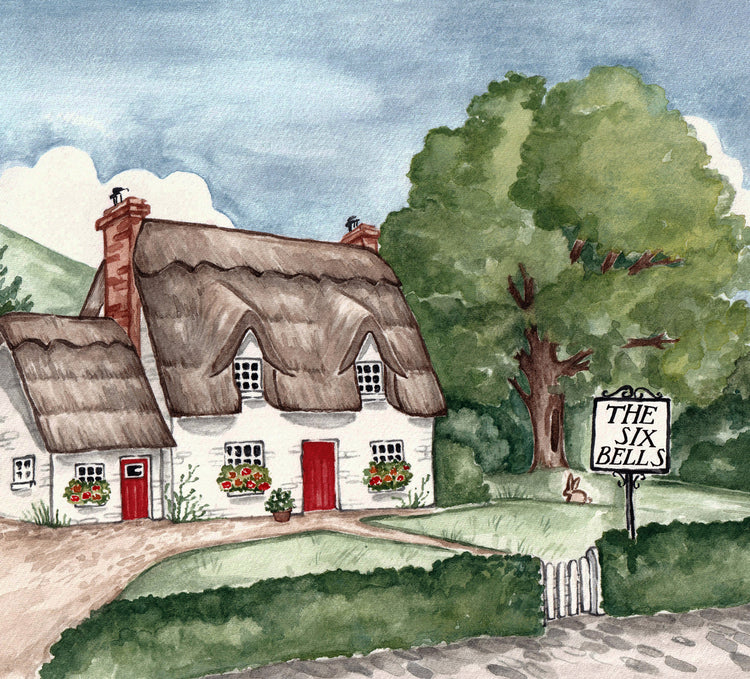This charming and quaint painting depicts a country house, possibly a farmhouse, rendered in what appears to be watercolor or a mixed medium. The main house is a two-story structure made of white brick and topped with a brown, thatched roof. This home features two chimneys, a red front door, and red flowers flourishing in planters beneath the three front-facing windows. To the left of the main house, a smaller one-story annex, perhaps a guest quarter, also has a red door and a few windows, sharing the same white brick walls and thatched roofing.

In front of the house is a green lawn, bordered by a white picket fence intertwined with a green hedge, separating the property from a brownish-gray walkway and driveway. A sign sticks out from the hedge, clearly reading "The Six Bells" in black letters. A rabbit can be seen on the lawn, adding to the idyllic country scene. 

In the background, to the right of the house, a large tree with abundant green foliage stands tall. Behind this tree, more green bushes can be seen, and above the entire scene, the sky is a light blue dotted with a few white clouds. On the left side, a green hill or mountain rises gently in the distance, enhancing the serene and picturesque setting of this delightful countryside property.